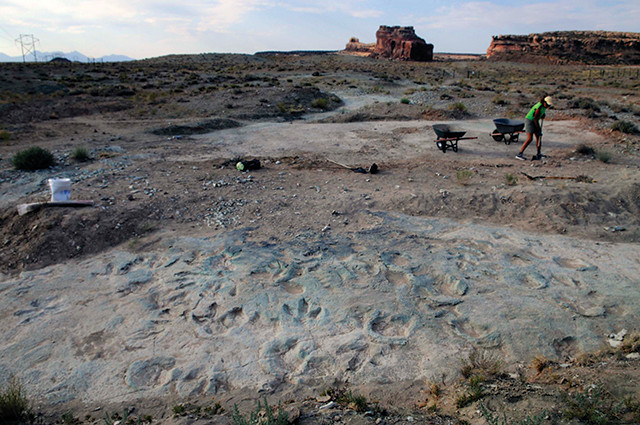The photograph depicts a rugged, desert-like canyon area characterized by a sandy and rocky terrain with scattered shrubbery and depressions that resemble animal hoofprints. Dominating the lower and central portions of the image is a person engaged in digging with a shovel or trowel, wearing sneakers, denim shorts, a green shirt, and a white baseball cap. Nearby, to the left, are two empty black wheelbarrows and a white plastic bucket. The background reveals rough, brown-colored rock formations, possibly part of a mountain range, stretching across the horizon. The blue sky above is partially adorned with white clouds and faint power lines in the upper right corner. The overall lighting suggests an early morning or late afternoon setting, adding a serene yet industrious atmosphere to the scene.